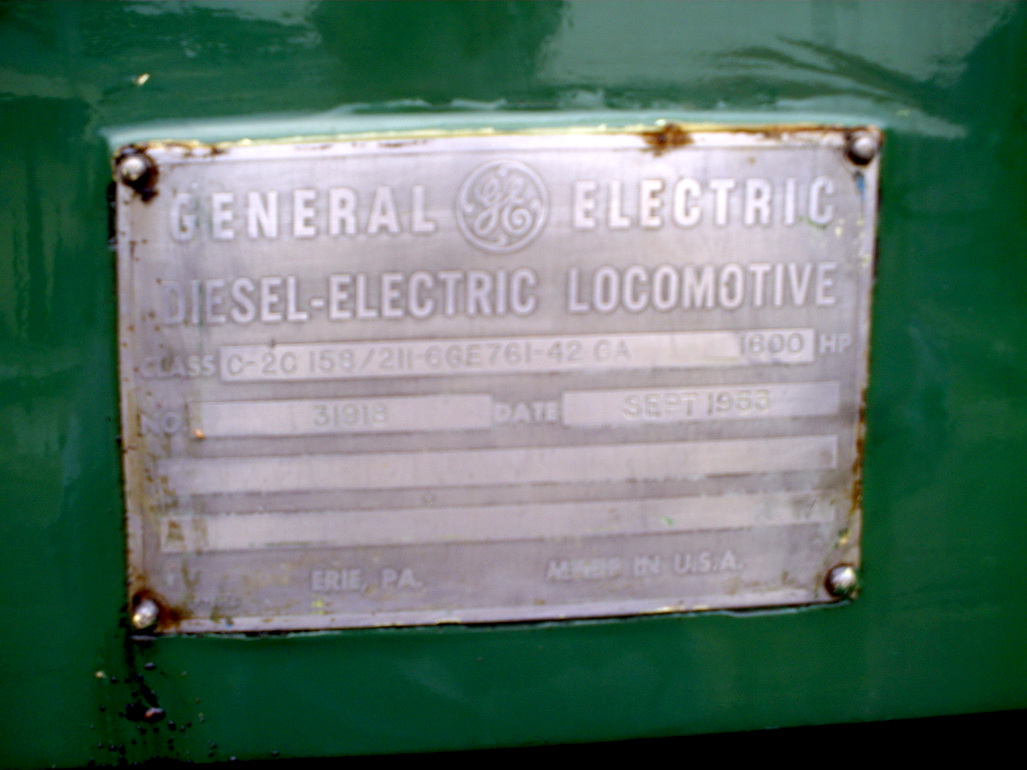This image features a rusted silver metal plaque affixed to a dark green metal surface, likely the end of a locomotive, using four corroded screws. The weathered sign bears significant fading, especially around the screws, with pronounced rust emanating from the lower-left bolt. The plaque reads "General Electric" at the top, with the GE logo centrally placed between these words. Below, it states "Diesel Electric Locomotive" followed by a class and model number: "Class C-2C1 5-8/2-1-1-6 GE 7-6 1-4 2 CA." Additional specifications include "1600 HP," a partial date which appears to be from 1953, and the manufacturing details "Erie, PA" and "Made in USA" at the bottom. Three sections on the plaque are left blank, and the metal edges show signs of significant rust and age.